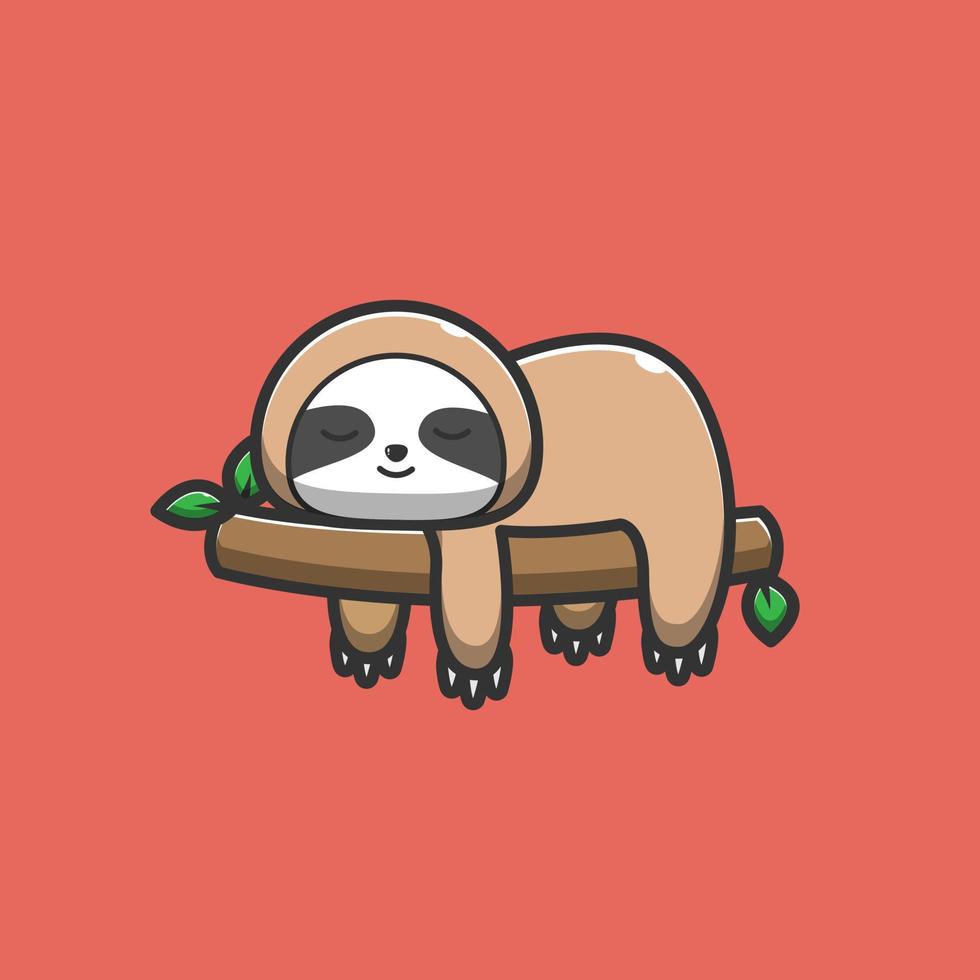The image is a cartoon drawing of a sloth, created using digital programs with a smooth and vectorized appearance. It features very thick black outlines and a light tan furry body. The sloth has a white face with black bands around its closed eyes, which are shaped in a smiling crescent expression. It has an oval body with four limbs draped downward, each ending in three white triangular claws. The sloth is laying across a slightly curved, brown log adorned with three green leaves—two on the top left and one on the bottom right. The background is a matte red, giving the overall image a light faded appearance with an orange-ish salmon pink hue. The sloth's shiny, almost blobby, cartoony shape contrasts against the simplistic, square-shaped backdrop, evoking a sense of serene contentment as it rests peacefully atop the log.